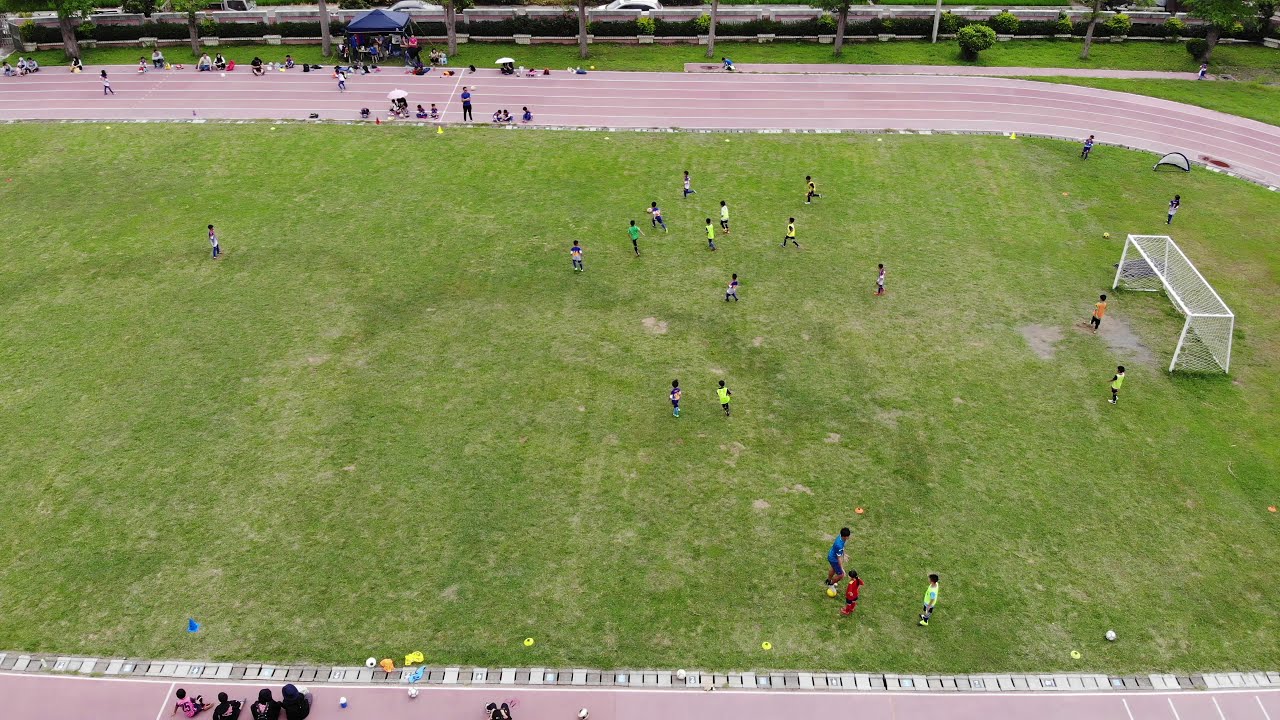This detailed aerial, landscape-oriented color photograph captures a lively youth soccer practice on a makeshift field set inside an oval, pink-colored track with distinct white striping. The drone photography offers a bird's-eye view, revealing numerous children in various uniforms of green, blue, white, red, and yellow scattered across the green grass, engaging in different drills rather than a single organized game. A white soccer goal sits prominently at the right side of the field, amidst neon-colored cones typically used for agility exercises. On the far left of the image, a blue pop-up canopy is visible behind some spectators seated on the track, with additional viewers dispersed at the top and bottom, likely parents or coaches. The sky is not visible, but umbrellas suggest preparations for either potential rain or sun protection, emphasizing the bustling yet casual atmosphere where families gather to watch the young players. Soccer balls and a few adults guiding the kids further enhance the scene's dynamic and instructional nature.